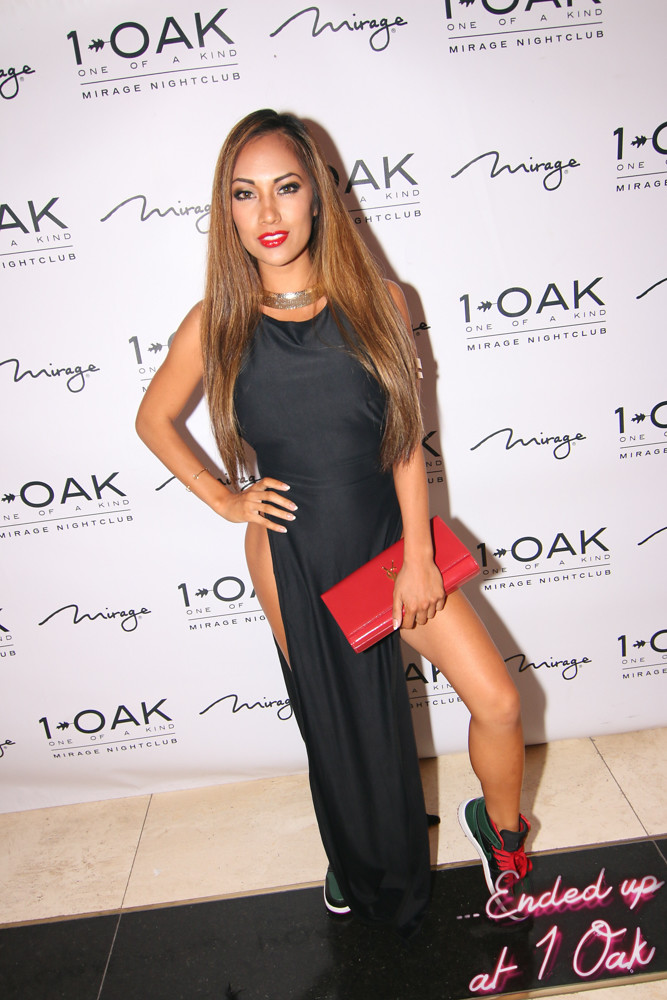This full-length color photograph captures a stylish young woman posing confidently at what seems to be an indoor event. She is wearing a striking sleeveless black dress with high slits on either side, revealing her legs and right hip. The dress is paired with gray sneakers featuring red laces, adding a casual twist to her ensemble. Her straight, honey-brown hair cascades down to her waist, and she complements her look with a thick gold necklace and bold red lipstick. In her left hand, she holds a red clutch, and she strikes a pose with her left leg bent and toe pointed, accentuating the dress's slits. The backdrop is a white wall adorned with company logos and the names "Mirage" and "One Oak," which appear multiple times in an alternating pattern, suggesting sponsors of the event. Notably, "ended up at One Oak" is written in playful pink neon letters at the bottom right corner of the image. The floor she stands on features a cream and black color scheme, further enhancing the photograph's stylish and modern aesthetic.